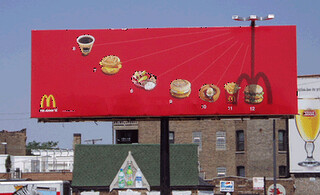This photograph features an elevated McDonald's billboard set against a clear blue sky. The billboard prominently displays the iconic yellow McDonald's arches in the lower left-hand corner. An innovative sundial device is integrated into the billboard's design, with metal arches positioned at the top. As the day progresses, the shadow from the arches shifts, highlighting different McDonald's menu items arranged from the top left to the bottom right. In the morning, the shadow points to a cup of coffee on the left, while by noon, it moves to highlight a burger at the bottom, ingeniously using natural light to emphasize different meal options throughout the day.